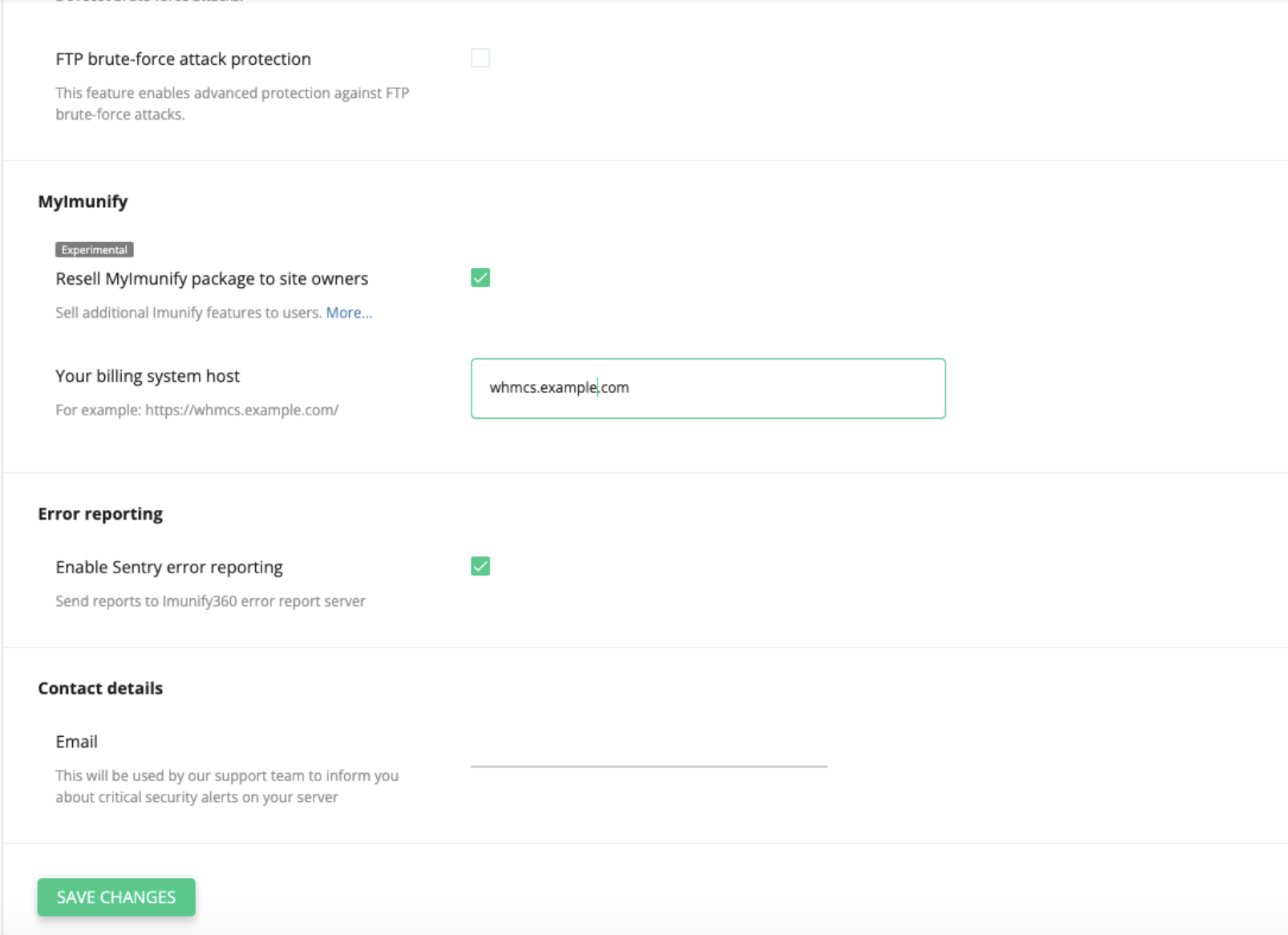The image displays a user profile settings page on a website, where various customization options are available for editing. The "My Immunifier" section stands out, requesting the user to input their email address. Directly below, there is an "error reporting" setting which can be toggled on or off. This option is highlighted in a green box situated on the right side of the page. Beneath the error reporting setting, users can input their contact details, also primarily their email, which is enclosed within a green border. Each category includes additional explanatory text written in gray, contrasting with the primary settings text in black. At the bottom left corner of the page is a "save changes" button, colored green with white text, ensuring that user modifications can be stored. The top of the image showcases a navigation bar with additional settings for further user customization.